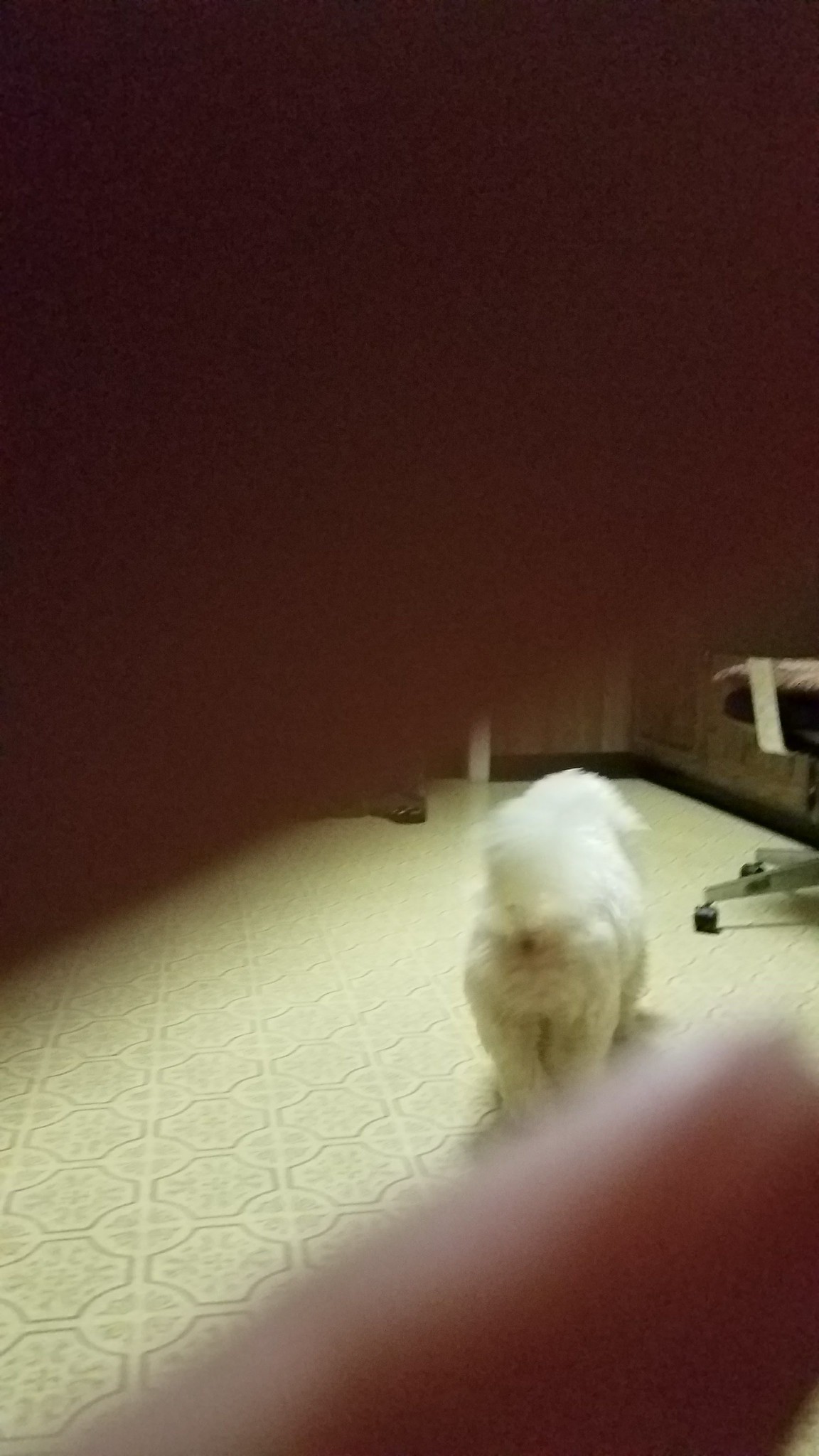The image is a vertically rectangular frame partially obscured by two fingers intruding into the shot—one covering almost the entire upper portion and another in the lower right corner. Between these fingers, a glimpse of tan, linoleum-like flooring with symmetrical designs is visible. Just right of center, a short and extremely fluffy dog is captured from behind, showcasing its elevated tail and furry posterior.